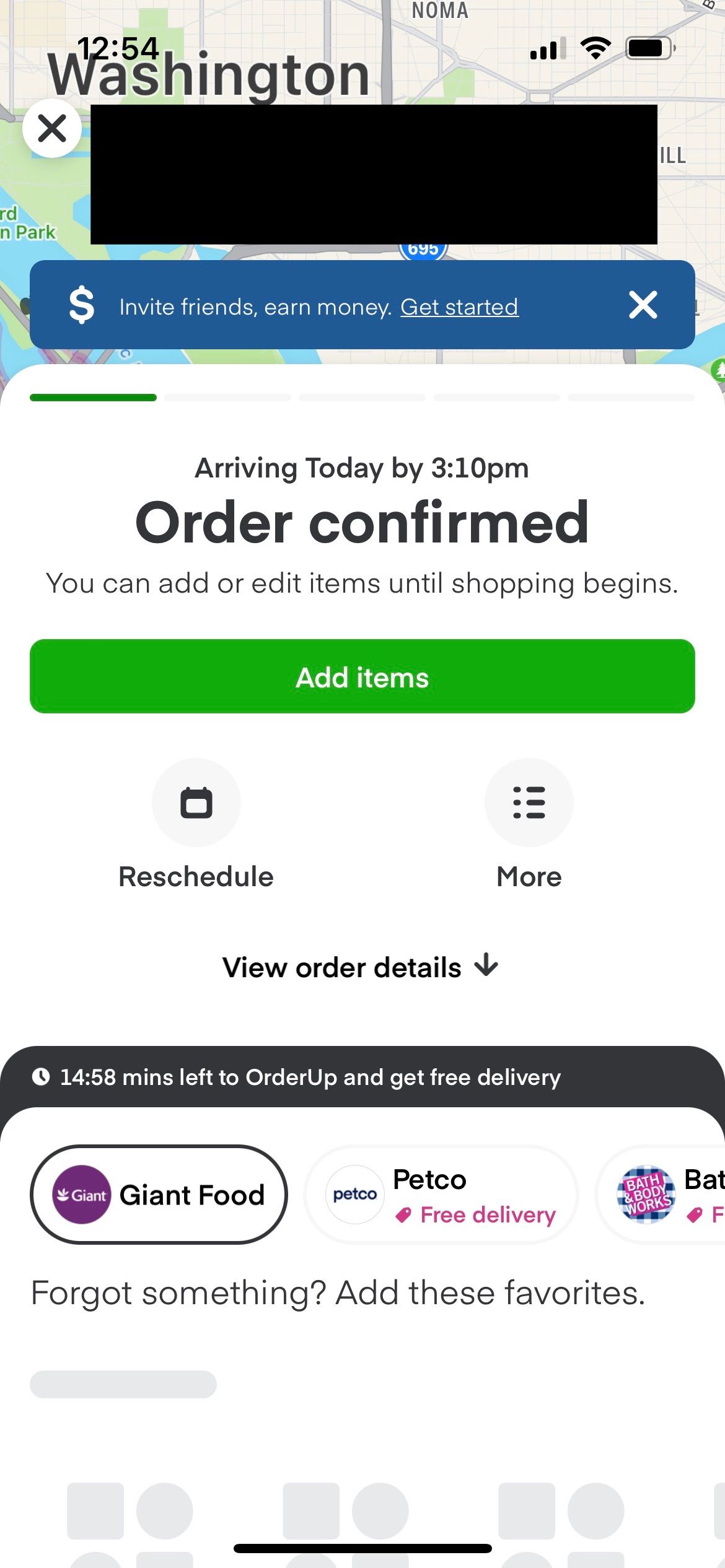The image depicts a smartphone screen displaying several app elements superimposed on a map of Washington. In the top left corner, the word "Washington" is prominently displayed in large black letters. Above this, the time is indicated as 12:54. The phone's status bar shows nearly full battery life and a strong connection signal.

Prominently featured is a large black box covering part of the map. Within this box is a white circle containing a black "X," below which there are options to "Invite friends, earn money, get started," displayed in a blue button with a dollar sign icon to the left and an "X" to the right.

An additional overlay appears above the map, revealing details about a delivery order. A progress bar indicating the delivery status is only partially filled, with text stating "Arriving today by 3:10 p.m. Order confirmed" in bold black letters. Users are informed that they can "add or edit items until shopping begins," accompanied by a green "Add items" button. Beneath this, there are options to "Reschedule" and a "View order details" button, indicated by a circle with three horizontal lines and a downward arrow respectively.

Further down, within a black outlined box, the text "14 minutes 58 seconds left to order up and get free delivery" is displayed, suggesting that users act quickly. Several delivery store options are circled, including "Giant Food" in gray and "Petco" offering free delivery. Part of the screen shows "Bat Mrs." and a prompt to "Add these favorites," though the text becomes unreadable towards the bottom where other gray images are visible but not legible.